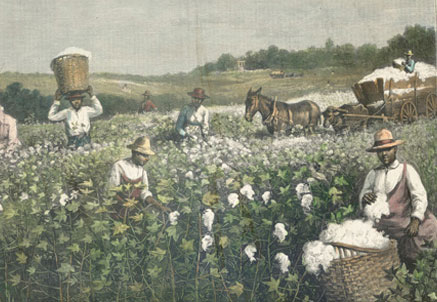The illustration is a rectangular painting depicting a historically evocative scene of African American slaves laboring in expansive cotton fields. The scene captures six workers, dressed in brown and white clothing, and wearing either tan or brown straw hats. Prominently, one man is discreetly balancing a large wicker basket brimming with cotton on his head, both hands steadying the hefty load. In the foreground, another man, donning a brown straw hat, clutches a substantial chunk of cotton towards the viewer, his oversized basket teeming with the fluffy yield beside him. Additionally, a loaded cart, pulled by two donkeys, anchors the scene towards the right. Curiously, a man sits amidst this pile in the cart, topped with cotton all around him. Stretching behind the workers is a lush green valley or meadow, seamlessly blending into a dense forest. The sky overhead is a somber grey, giving the image a poignant, timeless feel that echoes the enduring hardships of those depicted. This artwork, steeped in the cotton-picking heritage that Sellinger captures so compellingly, conjures a vivid glimpse into the arduous labor of the era.